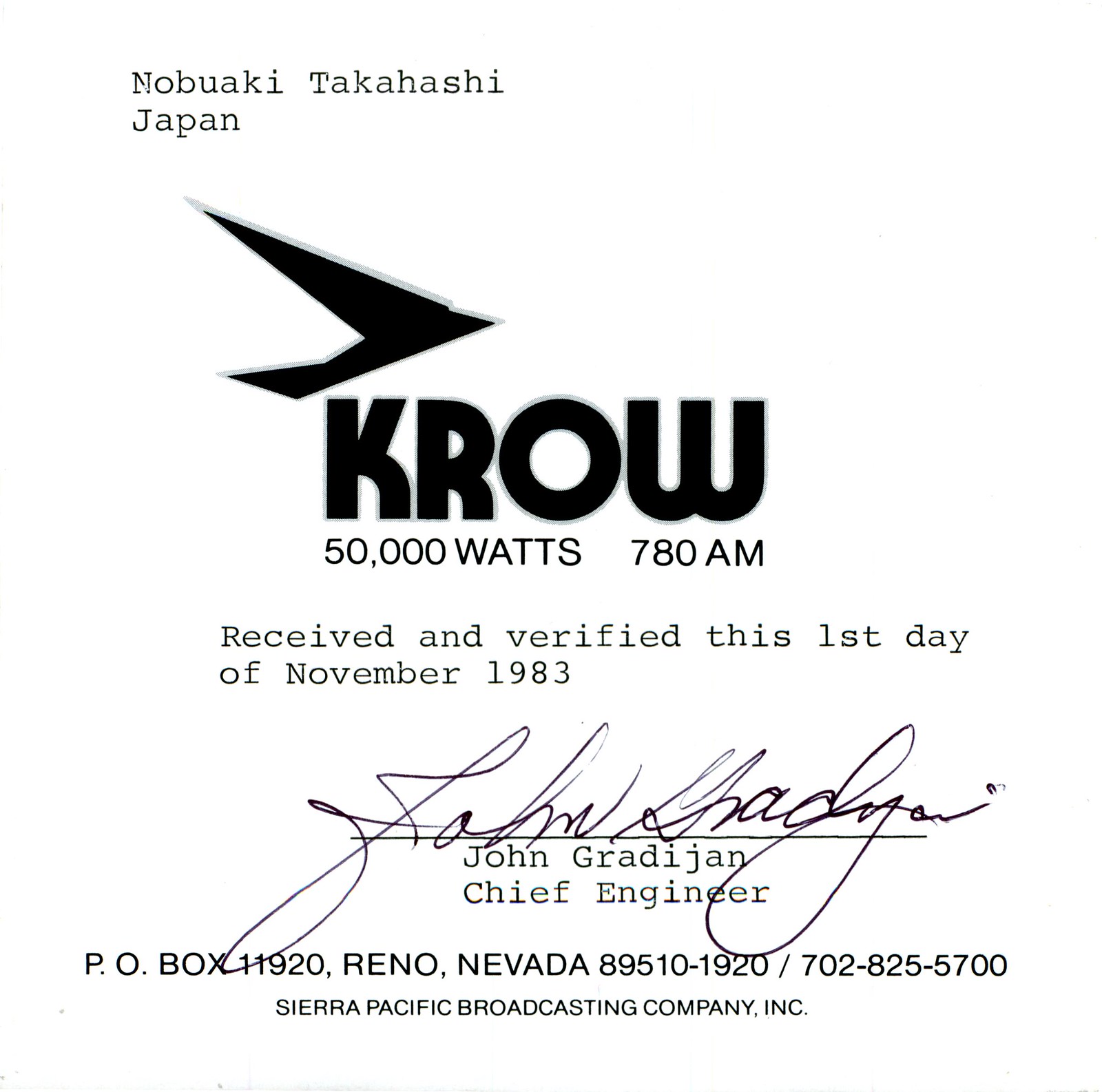The image depicts a verification letter sent to Nobuaki Takahashi from Japan. The top left of the letter features Takahashi's name and origin. Next to this, a logo resembling a wing or a bird, accompanied by the bold letters "KROW," indicates a radio station operating at 50,000 watts on 780 AM. The main body of the letter certifies that the signal was received and verified on the first day of November 1983. Toward the bottom is a handwritten signature in black ink from John Gratigen, identified as the chief engineer. Beneath the signature, the letter provides detailed contact information, including a P.O. Box address (P.O. Box 11920, Reno, Nevada, 89510-1920) and a phone number (702-825-5700), and it notes that the station is part of Sierra Pacific Broadcasting Company, Inc. The overall context suggests that this is a formal reception acknowledgment from the radio station.